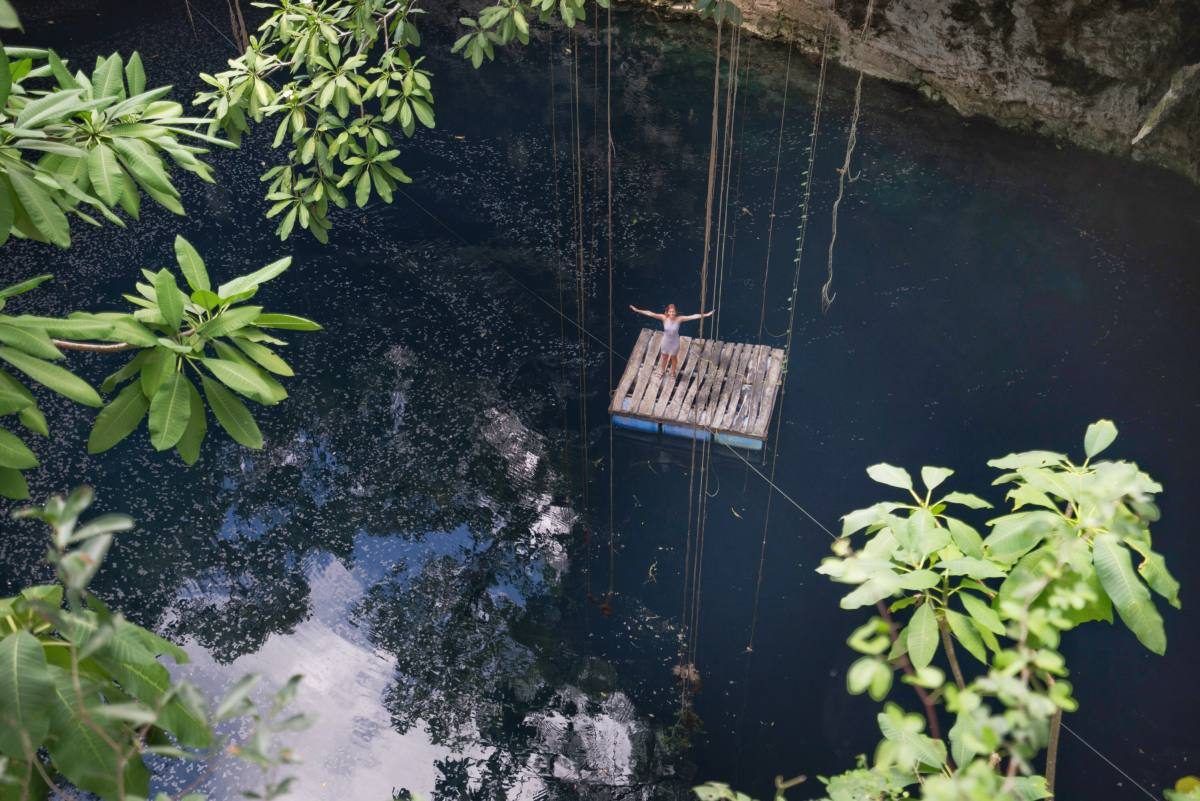In this highly detailed image, a woman in a white dress stands on a precarious, weathered wooden raft-like structure that appears to be suspended in mid-air over a mysterious, black-tinged body of water. She holds her arms outstretched in a T-pose, facing the camera from a distance sufficient to render her facial expression indistinct. The scene is enveloped in lush, vibrant tropical greenery with overhanging trees and vines, suggesting a jungle or rainforest setting. Numerous ropes and wires, potentially remnants of a broken bridge, dangle from above, intertwining with the wooden planks beneath her. Below and around her, the dark water churns with foamy waves, contrasting with the serene yet precarious ambiance created by the surrounding verdant foliage. The perspective of the photograph seems to be from a higher vantage point, looking down toward the woman, amplifying the sense of height and depth within the scene.